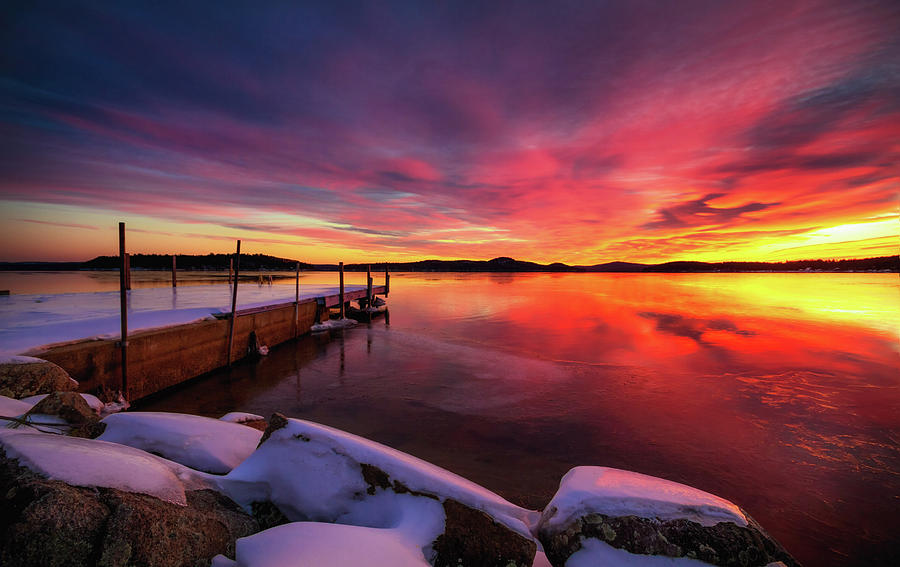This is a color photograph capturing a breathtaking sunset over a large body of water, possibly a lake or ocean, in a snowy landscape. The sky, adorned with wispy clouds, bursts with vibrant hues from the setting sun on the far right. There are rich pink, orange, and yellow tones near the sun that gradually transition to deeper reds, purples, and almost blackish tones towards the far left and top corners of the image. These stunning colors are beautifully mirrored on the still surface of the water below.

In the background, a series of dark hills or mountains stretch across the entire width of the image, their silhouettes adding depth to the serene scene. In the foreground, on the left side, stands a wooden pier or dock. This structure, with slanted poles on its sides, appears brown but is heavily laced with snow or ice. Further down to the left, there's a rocky border also cloaked in white ice, partially melted yet forming a thick, strikingly white layer. The composition of elements—the vivid sky, reflective water, dark hills, and icy foreground—creates a visually captivating and serene winter sunset scene.